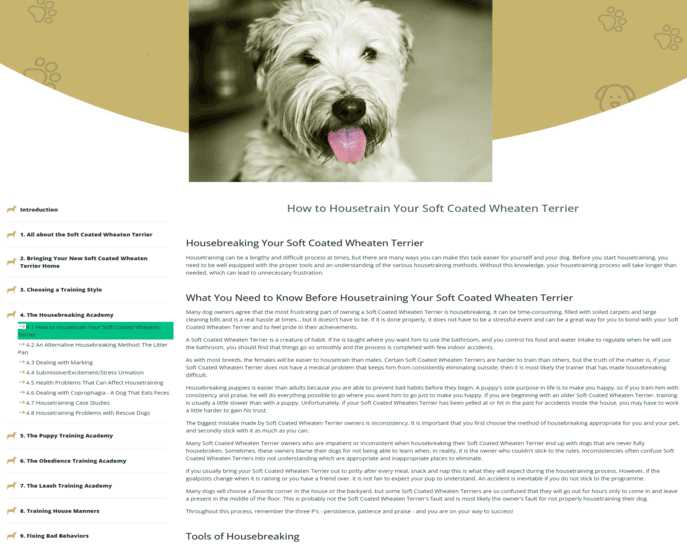The image is a screenshot taken from a web page dedicated to training Soft-Coated Wheaten Terriers. At the top of the page is a photograph of a small, white dog with a mix of gray fur on its face and body. The dog has expressive black eyes and its tongue sticking out, facing directly towards the viewer.

Below the image is the title of the website, "How to House Train Your Soft-Coated Wheaten Terrier." The web page is densely packed with information on various aspects of house training this specific breed. Some of the prominent section titles visible include "Housebreaking Your Soft-Coated Wheaten Terrier," "What You Need to Know Before House Training Your Soft-Coated Wheaten Terrier," and "Tools of Housebreaking." The page features extensive text with long sentences and paragraphs, suggesting detailed content.

On the left side of the page, there are different clickable sections listed as chapters, including "Introduction," "The Puppy Training Academy," and "The Obedience Training Academy," indicating a structured and comprehensive guide aimed at helping dog owners train their Soft-Coated Wheaten Terriers effectively.